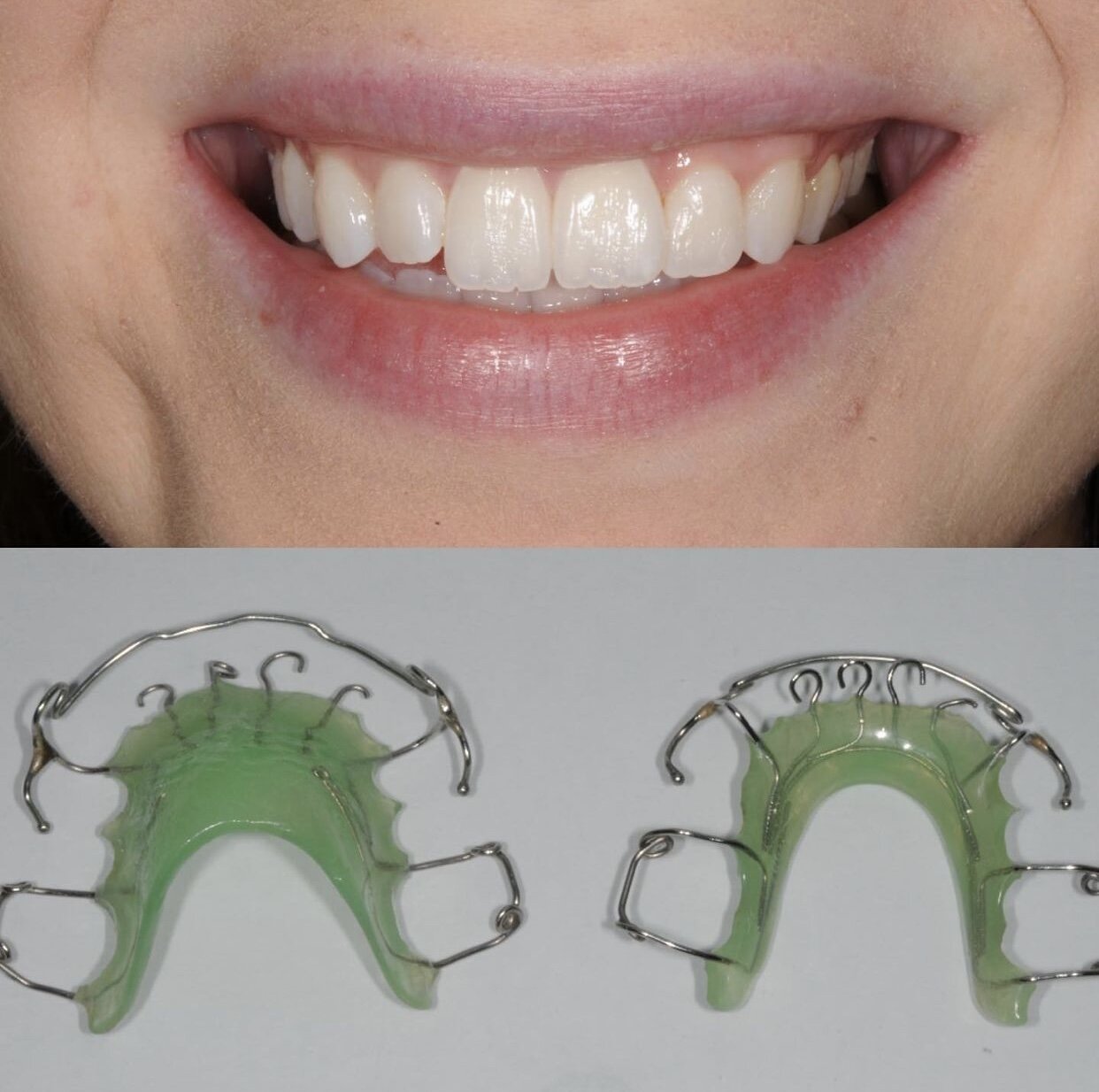This is a collage consisting of two photographs. The top horizontal image features the lower half of a young lady’s face showcasing her wide, radiant smile. Her teeth are notably straight and clean, a testament to effective dental work. The focus is clearly on her well-aligned, organized set of teeth. Below this, the second photograph displays two similar green dental retainers side by side on a smooth gray background. These retainers have transparent green acrylic sections with intricate metal components designed to fit within the mouth, facilitating the teeth-straightening process. The combination of these photographs illustrates the transformative journey of achieving a perfect smile through diligent orthodontic treatment, emphasizing the role of the retainers in straightening her teeth.